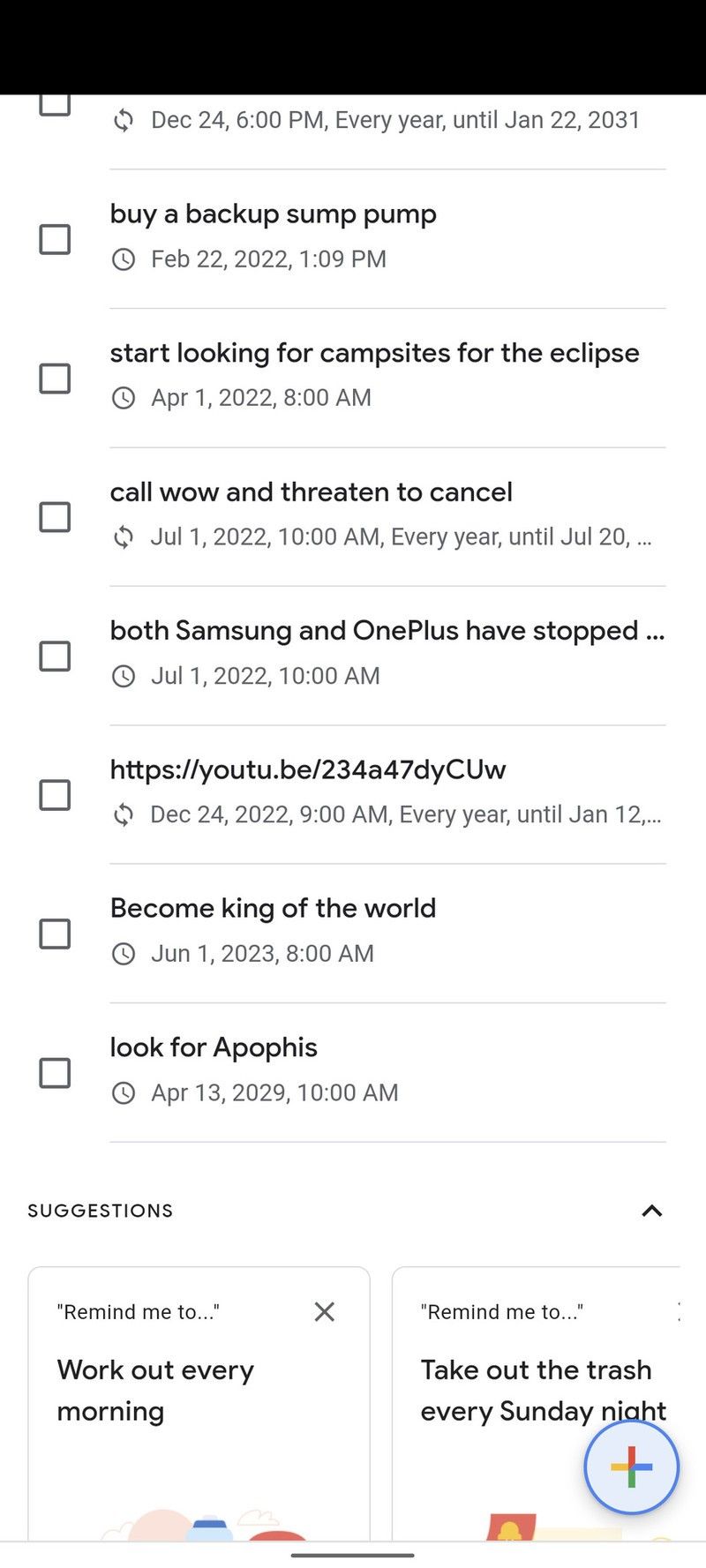Here's a cleaned-up and detailed caption for the image based on your description:

---

A visually cluttered screenshot of a digital task list with various reminders and notes. The list includes a range of tasks with specific dates and times:

1. **Buy a backup sump pump** - February 22, 2022, at 1:09 PM.
2. **Start looking for campsites for the Eclipse** - April 1, 2022, at 8:00 AM.
3. **Call to cancel a threat** - July 1, 2022, at 10:00 AM.
4. **YouTube URL** - December 24, 2020, at 9:10 AM.
5. **Become king of the world** - June 1, 2023, at 8:00 AM.
6. **Look for a pop-up** - April 13, 2029, at 10:00 AM.

The image also features suggestions, indicated by an arrow pointing upward. Two checkboxes appear beside the suggestions: one to remind the user to work out every morning, and the other to remind them to take out the trash every Sunday night.

In the bottom right-hand corner, there is a circular icon with a rainbow "+" symbol inside it. The bottom part of the image displays a multicolored graphic, although it is partially cut off.

Overall, the image showcases a densely packed schedule with a mix of personal reminders, ambitious aspirations, and routine tasks.

---